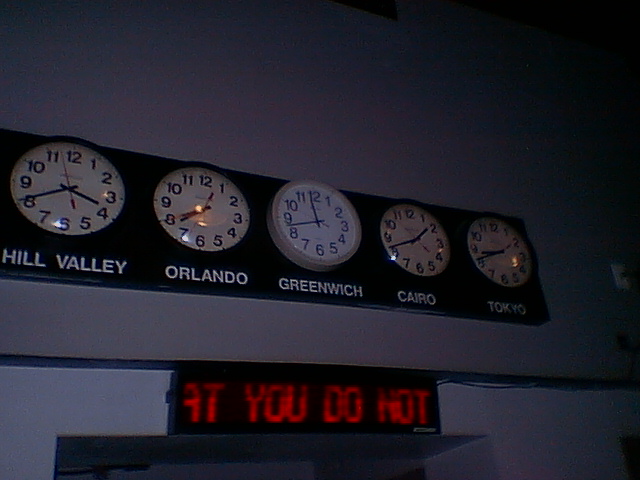In this dimly lit photo, illuminated by a camera flash, we see a horizontal arrangement of five clocks mounted on a sleek black rectangle of either plastic or metal. These clocks, positioned against a flat gray wall near the ceiling, each display the local time for different cities and feature uniform designs with white faces, black hour and minute hands, and a red second hand. From left to right, the cities indicated beneath the clocks are Hill Valley, Orlando, Greenwich, Cairo, and Tokyo. Each city's name is presented in black plastic capital letters. The four outer clocks are black plastic analog models, while the clock representing Greenwich is distinct with its gray plastic frame. Below this display, a rectangular ticker sign with red lettering reads "at you do not," appearing to be part of a larger scrolling message. Located in the lower right corner of the ticker is a small logo resembling a doorway, suggesting the entire setup is situated above an actual doorway in the building.